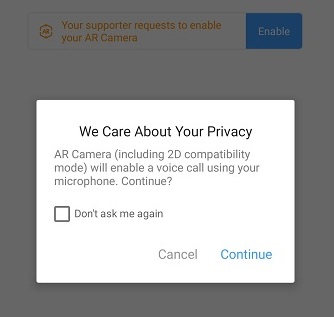This image is a screenshot of a prompt window. The prompt consists of a completely gray background with a header at the top. The header reads "Your supporter requests to enable your AR camera," and it doubles as an action button. This action button has a white background with orange text, and next to it, there's a blue button labeled "Enable."

Below the header is a white rectangular box with a clear message in black bold text, "We care about your privacy." Beneath this, more information is provided in gray text: "AR camera, including 2D compatibility mode, will enable a voice call using your microphone. Continue."

At the bottom, there is a checkbox option for users to select if they do not want to see this prompt again, labeled "Don't ask me again." In the lower right corner of the prompt, there are two clickable options: "Cancel" in gray text and "Continue" in blue text.